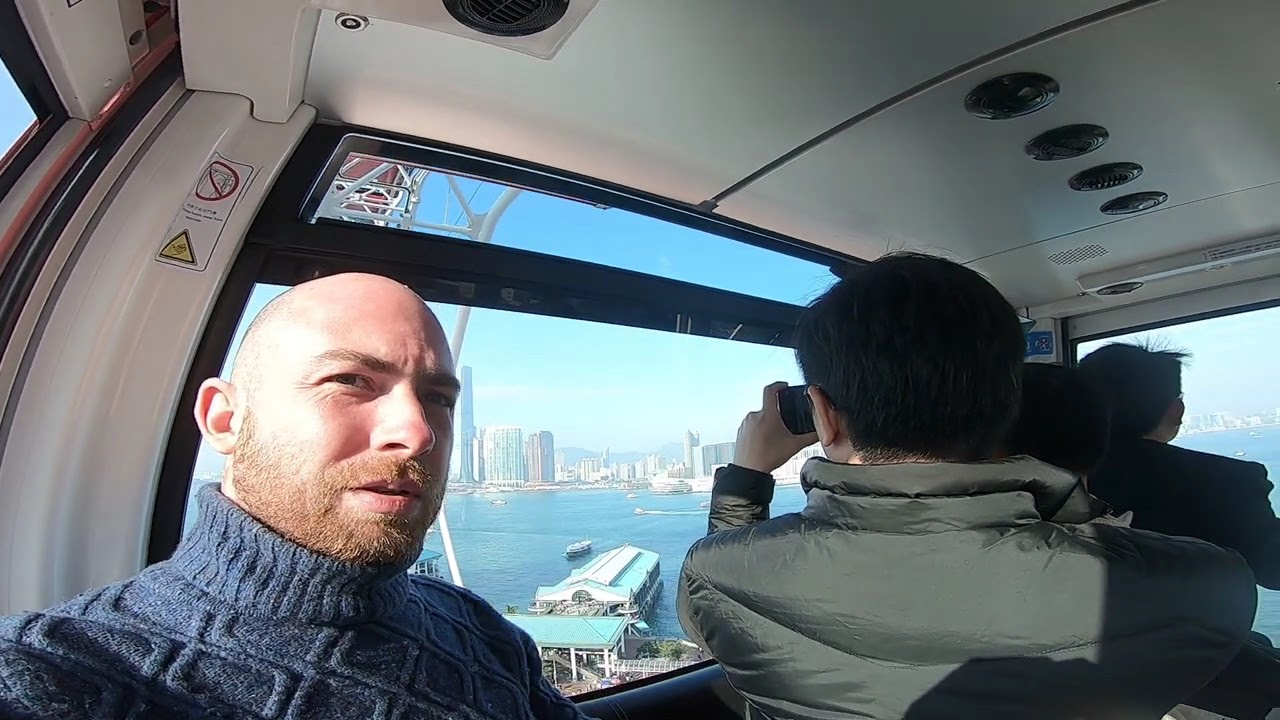The image captures a scene inside a compact, helicopter-like vehicle overlooking a city skyline, quite possibly New York City. The vehicle is high above the city, providing a stunning view of skyscrapers, a river, and a ferry navigating through the water. Inside the vehicle, on the left, a bald man with a red beard and blue cable-knit sweater looks directly at the camera. Next to him, a younger man wearing a jacket is absorbed in taking a photo with his smartphone, capturing the scenic cityscape outside the window. At the front of the vehicle, the driver, a man in a black suit with short black hair, is focused on navigating. A woman in a formal blazer is also present, possibly giving a tour or assisting with navigation. The scene suggests a specialized tour or a high-end commuting service, providing a detailed and intimate look at the city's aerial beauty.